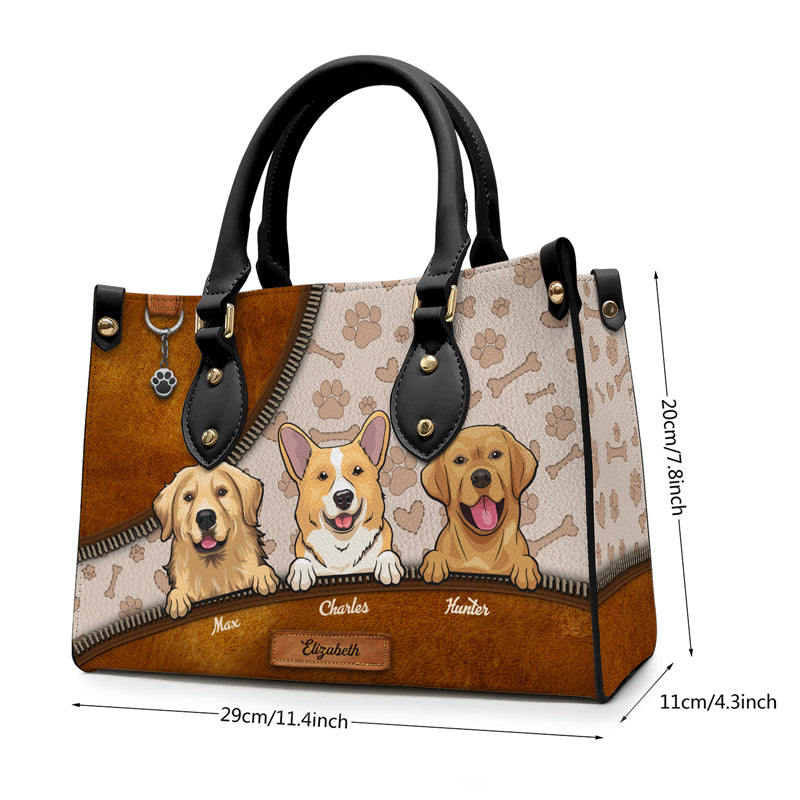This image features a luxurious square-shaped handbag, likely customizable and listed on a platform like Etsy. The handbag is crafted from high-quality leather and adorned with animated cartoon illustrations of three different dogs, named Max, Charles, and Hunter, whose tongues are out and appear to be smiling. Surrounding the dogs are playful patterns of bones and paw prints. The bag has two sturdy black leather handles and gold pins accenting its structure. On the upper section, there is a plain leather patch with a paw charm, adding to its detailed design. The handbag also prominently displays its dimensions for length, width, and height, and features a customizable leather label at the bottom that reads "Elizabeth."